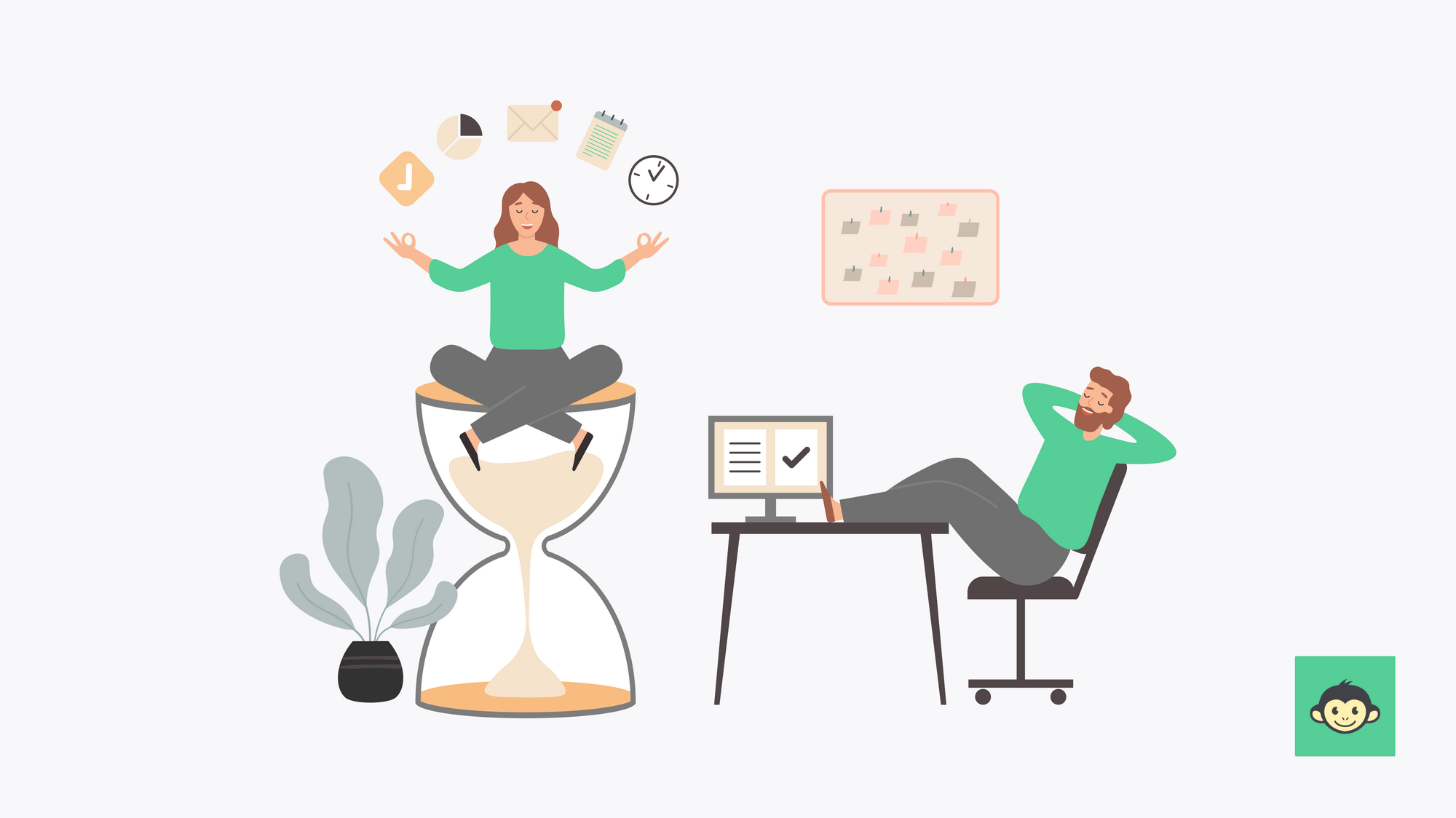This digital rendering portrays a detailed scene set in an office with a grayish background, highlighting the contrasting roles and activities of two cartoon characters. On the right side, a man with reddish hair and a full beard is reclining in a swivel chair, his feet propped up on a desk and his hands behind his head. He is dressed in a green pullover shirt and black pants. In front of him on the desk is a computer monitor displaying a large check mark, emphasizing a task completed or a goal achieved. On the wall behind him, there is a decorative plaque adding a touch of detail to the setting.

Contrasting sharply, in the center of the image, a woman also dressed in a green top and black pants is perched cross-legged on top of an hourglass. She strikes a yoga pose, fingers poised with thumb and forefinger together, embodying a sense of balance despite the task-laden environment around her. Above her head, she juggles a variety of items including a clock, mail, and check marks, symbolizing the multitude of duties she is managing. To her left, a plant in a black pot with gray leaves adds a touch of greenery to the office scene.

In the lower right corner of the image, a green square displays a picture of a monkey, potentially serving as the artist's signature or a playful element within the illustration. The overall imagery vividly contrasts the man's relaxed demeanor with the woman's active multitasking, perhaps offering a commentary on gender roles or the daily realities faced by women.